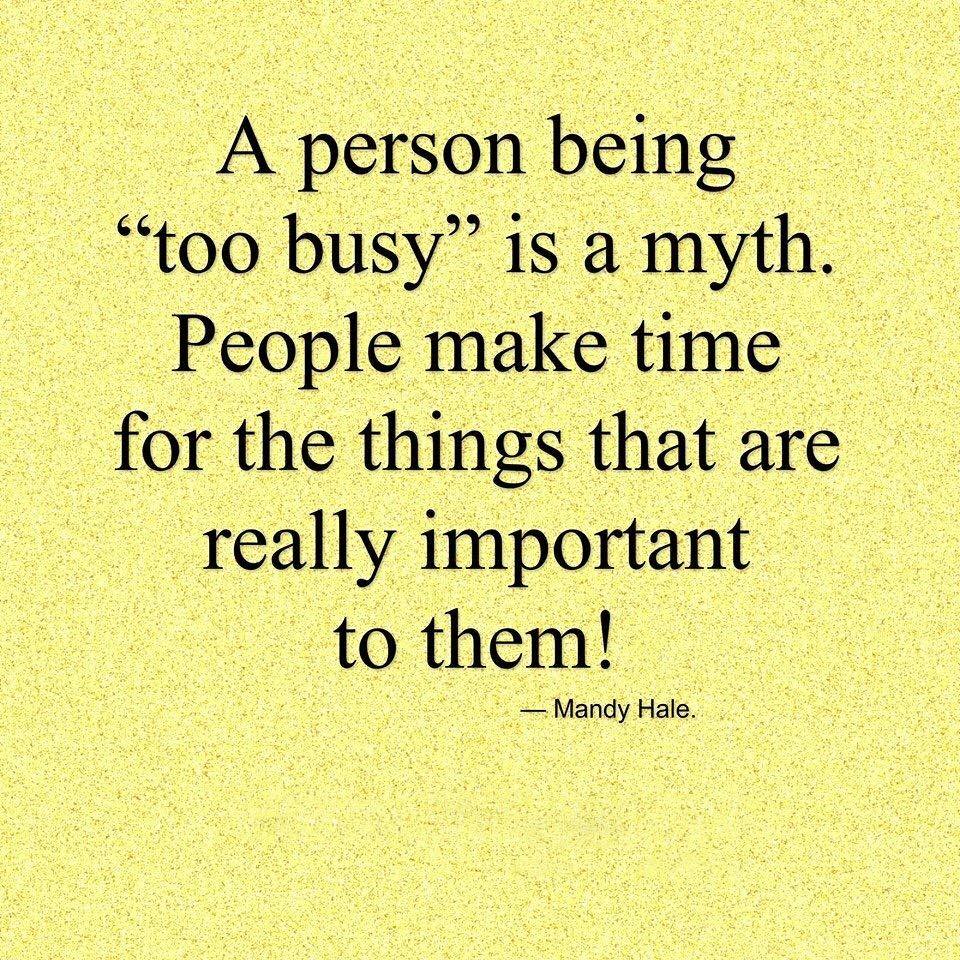In the image, a motivational quote is displayed on a background that features multiple shades of yellow with gray and brown specks, creating a static-like effect. The black text is centered in the upper portion of the image, with a noticeable empty band along the bottom. The quote reads, "A person being 'too busy' is a myth. People make time for the things that are really important to them!" Following the main text is the attribution, "Mandy Hale." The overall style and setting suggest it is an inspirational message commonly found on social media. There are no other objects or images present.